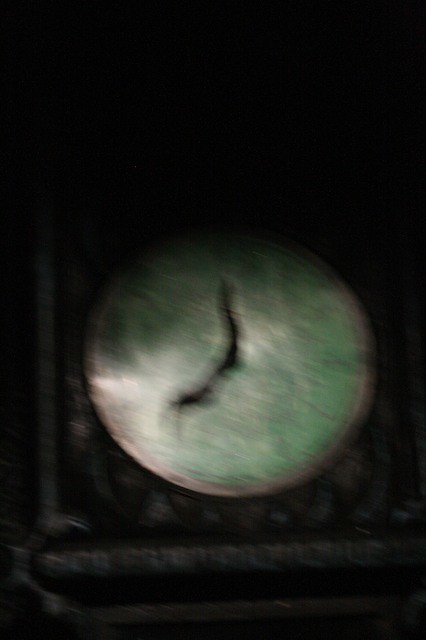This blurred and pixelated photograph presents a perplexing, abstract image that is difficult to interpret. Dominating the center of the image is a white element resembling a button or a disc, featuring a simplistic smiley face – merely a curved smile without eyes – which lends an enigmatic, almost whimsical aura to the picture. This white smiley disc stands out against a dark, perhaps black background. Around this central figure, there are a couple of distinct lines, one forming an L-shape and the other running vertically.

Further examining the image, one notices a green disc, possibly made of stone like jade, encased in a gray-colored metal frame. This green disc seems to be mounted within a larger structure resembling a square or rectangular frame. Some interpret this green disc as part of a larger clock face, featuring black hour and minute hands. The clock, likely analog, has a white face with indecipherable numbers or numerals, set within an ornate, wood-carved square backing that evokes the style of a grandfather clock.

Despite the varied interpretations, the consensus agrees on a central white smiley disc amidst a complex, dark background with additional shapes and forms contributing to an overall mysterious and abstract composition.